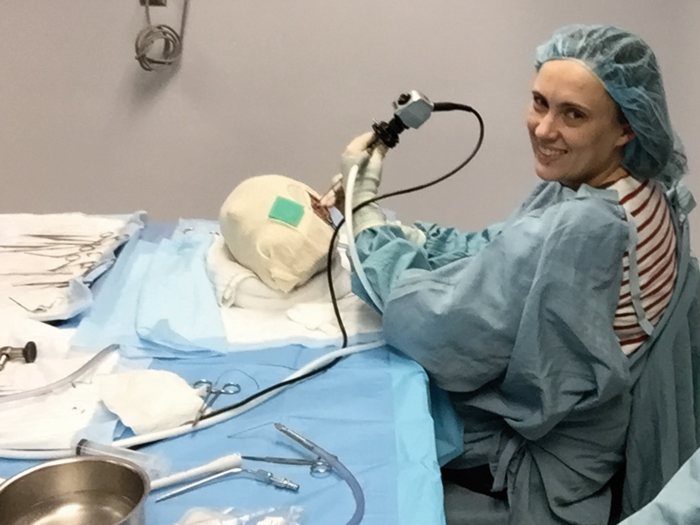The photograph depicts a Caucasian woman smiling at the camera, dressed in blue medical scrubs with a matching hairnet, and white gloves. Peeking out from under her scrubs is a white and red striped shirt. She is positioned in a setting that resembles a medical office, standing in front of a table covered with blue medical cloth. The table is cluttered with various surgical instruments including scissors, forceps, and clamps, along with a stainless steel pan and a metal bin. A black wire stretches across the table, which also has a green and brown patch that resembles an opened section of some non-living object, possibly a medical training device or model, rather than a person or animal. Behind her is a gray wall and a hanging wire, further emphasizing the clinical environment. She appears to be either handling or measuring the object with a tool, but the absence of a close-up shot makes her exact activity unclear. The setting appears informal and unposed.